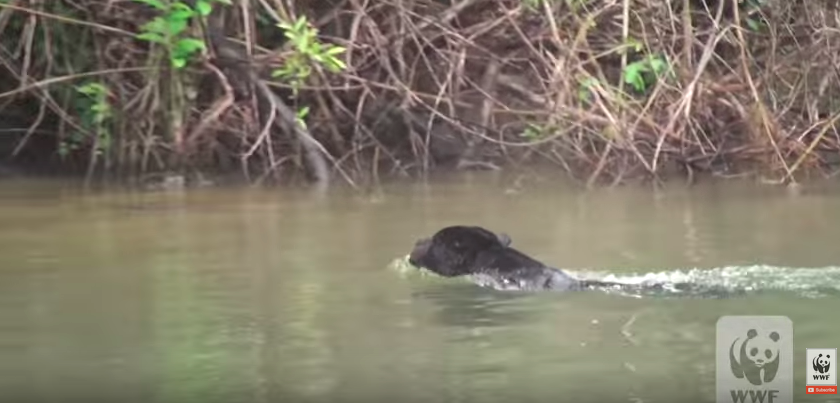The photograph captures a bear swimming in murky, muddy water, with only its head visible and facing away from the camera. The water, a mix of browns, dark greens, and dark yellows, dominates the lower half of the image, while the top half is densely packed with brambles, twigs, branches, and some green leaves. A wave of white water trails behind the bear, suggesting movement towards the shore. In the bottom right corner, there is a translucent WWF logo featuring a panda, alongside a white square containing another panda image with the text "WWF" and an unreadable red line above. The scene indicates a possible river or lake, not an ocean, and the overall impression is one of natural wilderness.